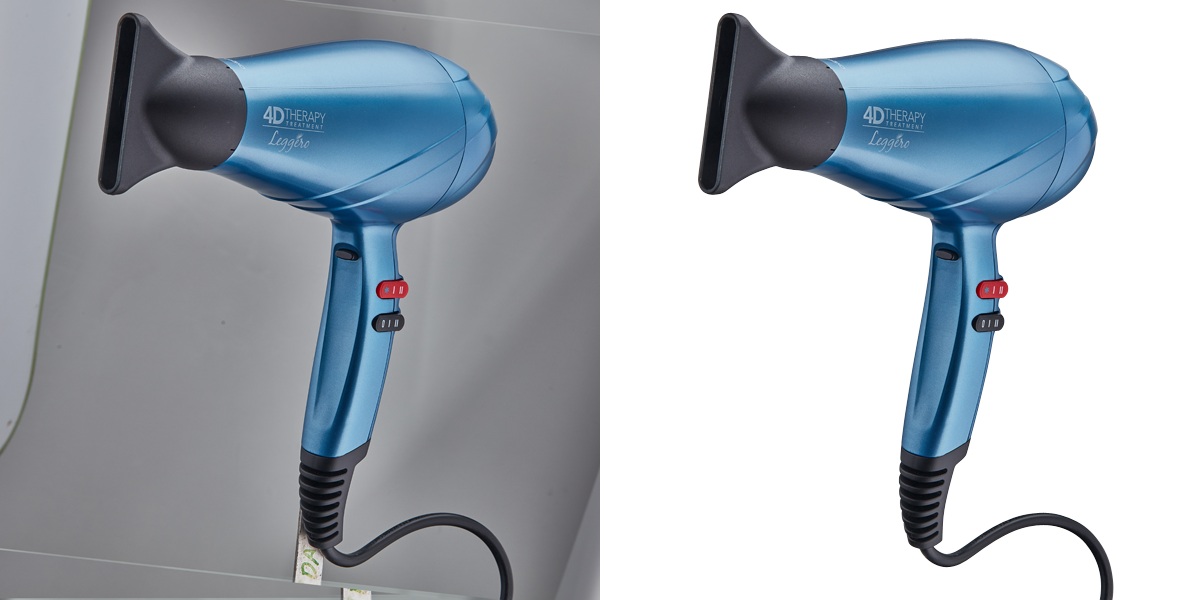This image showcases two side-by-side photographs of the same bright metallic blue hairdryer, both labeled with "4D Therapy Treatment." The hairdryer features a black cord, a black concentrator nozzle attachment at the end, and three buttons—all located on the handle: one red button and two black buttons. The photograph on the left presents the hairdryer resting on a gray bag against a gray, possibly leather, background. A small, partially visible tag on the bag reads "D.A." The photograph on the right depicts the identical hairdryer on a clean, white background. The model name "Leggere" is indicated on both hairdryers.